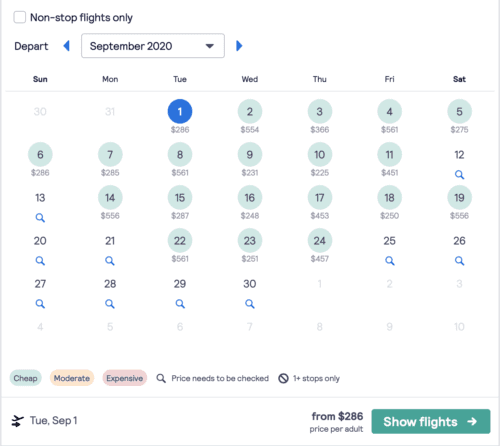Screenshot Description: Travel Date Selection Page

This image captures a screenshot of a travel webpage designed for selecting travel dates. The background is predominantly white, establishing a clean and organized interface. The format of the page resembles a calendar layout, indicating the user has navigated to the section where departure dates are chosen.

At the upper left corner of the page, there is an option labeled "Non-stop flights only" accompanied by a clickable checkbox. Directly beneath this option, the word "Depart" is displayed with an adjacent box set to "September 2020," featuring a dropdown menu allowing users to select the desired year.

The central portion of the page hosts a monthly calendar organized from Sunday to Saturday using standard day abbreviations. The calendar grid begins on Tuesday, September 1st, prominently marked with a blue circle, indicating the selected departure date. This date also shows a fare of $286. All other dates from the 1st to the 30th of September are encircled in green, each displaying a respective price.

Below the calendar, small buttons for filtering flight options—labeled "Cheap," "Moderate," and "Expensive"—provide additional user customization. A search box is available for further queries. Towards the bottom of the page, a conspicuous "Show Flights" button invites users to view available flights based on the selected criteria, clearly indicating a starting price of $286 per adult.